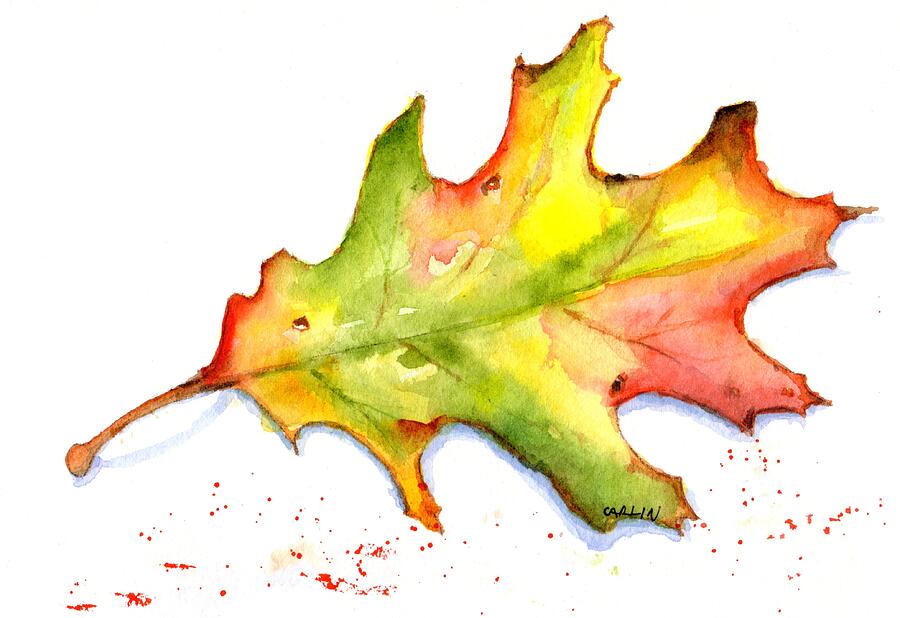This detailed watercolor painting, set against a clean white background, captures the essence of an autumn maple leaf. The leaf, predominantly facing to the right, exhibits a brilliant mix of reddish, orangish, yellowish, and greenish hues. The watercolor technique gives it a fluid and soft appearance, with the colors blending seamlessly together, which enhances its stylized, hand-painted charm. 

The stem, thin, curved, and predominantly orange, points to the left, contrasting slightly with its brownish-red shadow that suggests a three-dimensional quality. The shadow beneath the leaf adds depth, accentuated with an opaque purple hue.

Beneath the leaf, splashes and dots of red and yellow paint create a lively texture. The painting's bottom section, particularly where the green tones become prominent, features the artist's signature, "CARLIN," clearly inscribed in black ink, adding an authenticated touch to this vibrant depiction of nature.